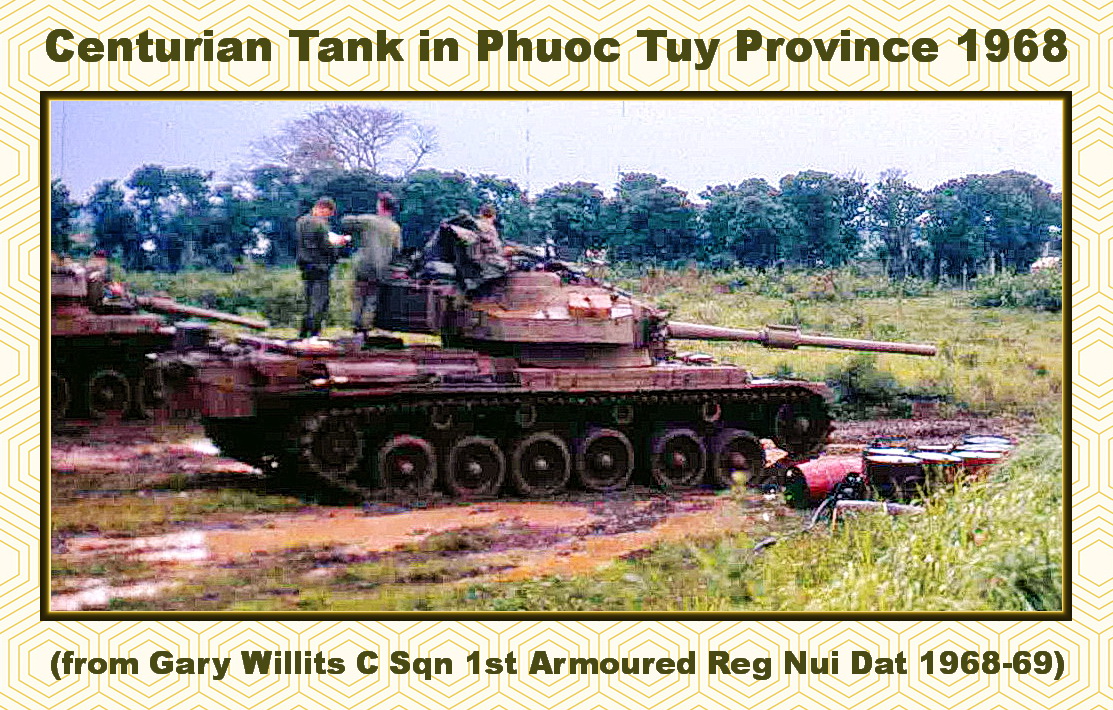The image portrays an old, color photograph with a vintage filter and a black border on a light yellow background. The top of the photo features green text reading, "Centurion Tank in Phuoc Thuy Province, 1968," while the bottom reads, "From Gary Willits, CSQN, First Armored Reg., Nui Dat, 1968-69." The setting is a muddy marshland, indicative of heavy rain, surrounded by tall grass and a backdrop of trees. At the center stands a Centurion tank with three men in green army uniforms, one in the turret seat and two behind it. Red canisters are visible in the foreground, along with another partial tank to the left with a single occupant, reinforcing the military context likely associated with the Vietnam War era.